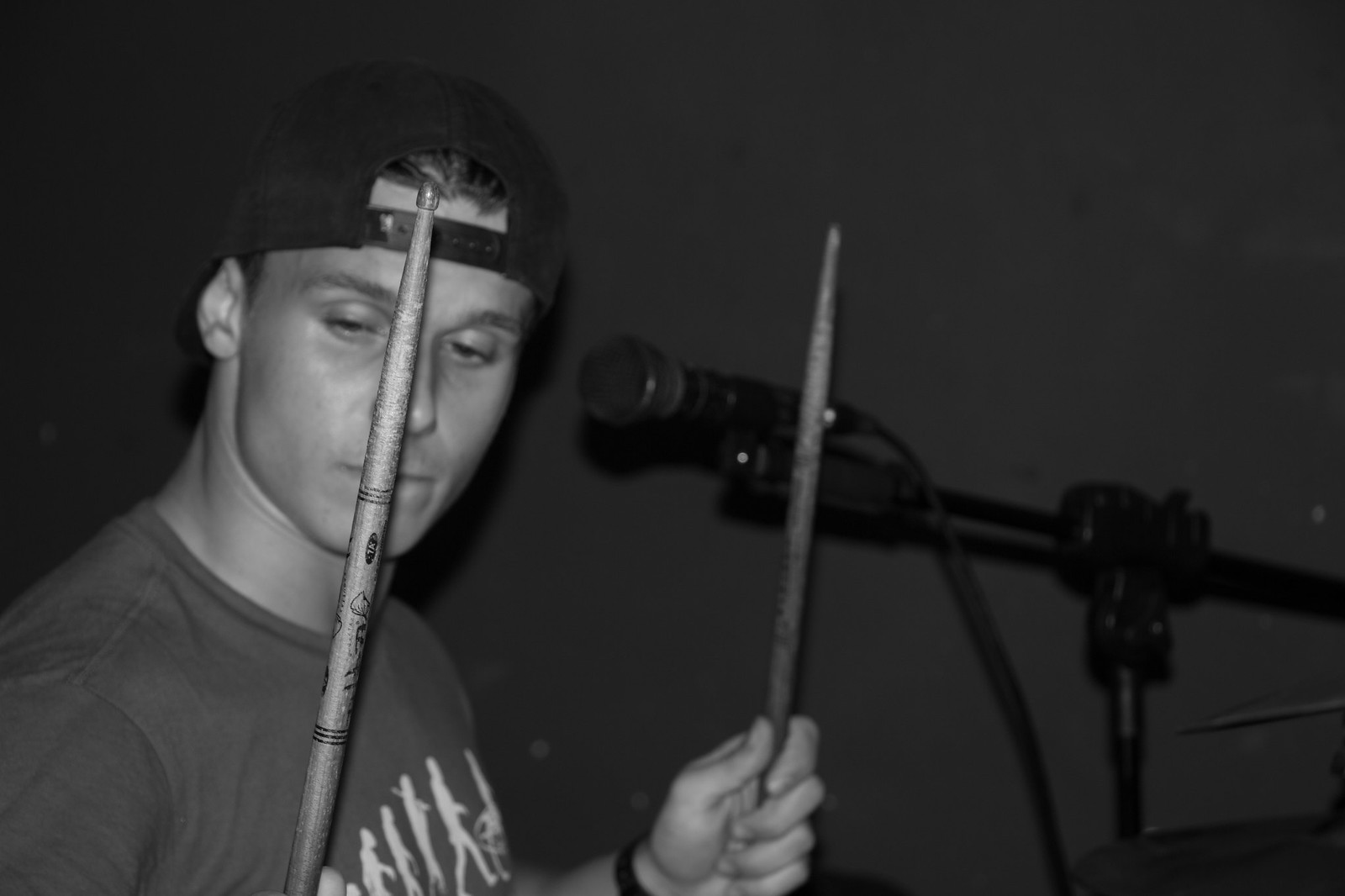This rectangular, horizontally-aligned, black-and-white photograph features a close-up of a drummer's face. The image is slightly blurry and depicts the drummer wearing a backward black ball cap and a t-shirt that has graphics illustrating the evolution of man—from an ape to a fully upright human. His expression is neutral, and he is looking slightly to his right and downward.

In the photograph, he is holding a drumstick in each hand. The drumstick in his right hand is vertically aligned, bisecting his face right between his eyes. The left hand and the drumstick it holds are also visible, positioned towards the right side of the picture (his left, the viewer's right). He's wearing a wristwatch on his left wrist.

The background appears to be a solid wall, darker in the upper left corner, creating a stark contrast with the lit-up face. Two microphones with black handles and visible tips are positioned in front of him, with one pointing towards his mouth. Slightly visible to the side are elements of his drum set, including a snare drum and cymbals.